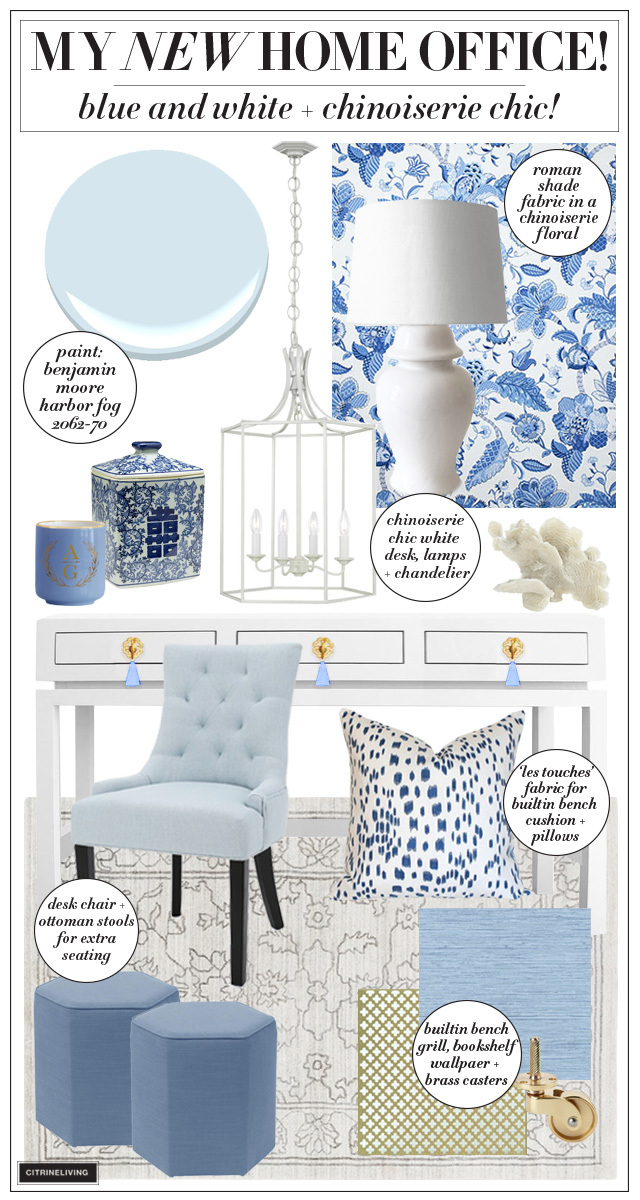The image is a four-panel advertisement for a new home office design, themed "My New Home Office: Blue and White, Chinoiserie Chic." At the very top, the title is displayed in black text on a white background, with an elegant script underneath. 

The upper left panel features a jar next to a clear glass container, likely a perfume bottle, set against a white background. Below this, there is a label for "Roman Shade Fabric in Floral." The upper right panel showcases a white lamp on a blue leafy background with white flowers beneath it.

In the center of the layout, there is a hanging glass chandelier labeled "Chic White Desk Lamps and Chandelier." Adjacent to this, the middle section highlights the paint color "Benjamin Moore Harbor Fog 2062-70" alongside two stylish vases.

The lower left panel displays a white cushioned chair with wooden legs and armrests, next to blue ottomans and a white pillow with blue spots, all set on patterned flowery wallpaper. To the right, the lower right panel presents additional decor: a white lamp, more pillows—including a blue and white checked one—and an assortment of white and brown checked cushions.

The overall aesthetic blends plush comfort with a clean, sophisticated look, featuring an array of coordinated blue and white decorative items, meticulously arranged to convey a cohesive and stylish home office design.